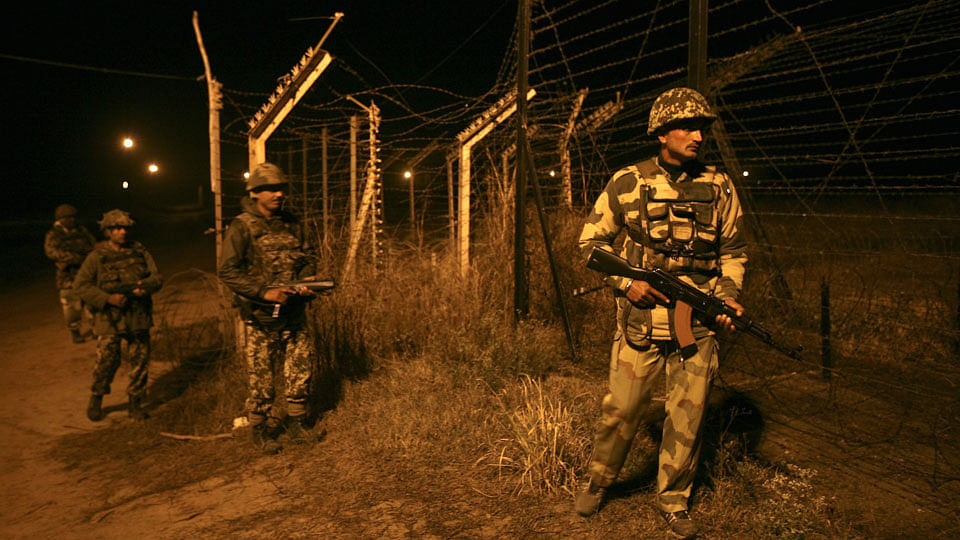In the nighttime image, four soldiers are patrolling alongside a wired fence with barbed wire, possibly at a military compound. All of them are clad in camouflage uniforms and helmets, and they carry various types of firearms, including what appears to be high-powered rifles. The soldier closest to the viewer, positioned on the right, is fully illuminated by an amber-colored light and can be seen holding a black rifle with brown handles. This soldier is distinctively more visible than the others due to the lighting, which suggests that they are standing directly under a low-level light source. The remaining soldiers, who seem to be standing or walking slightly behind him, have darker camo and their firearms are less clearly defined. The ground is covered with sparse short grasses, and the pitch-black sky, coupled with distant lights, indicates that the scene is set at night.